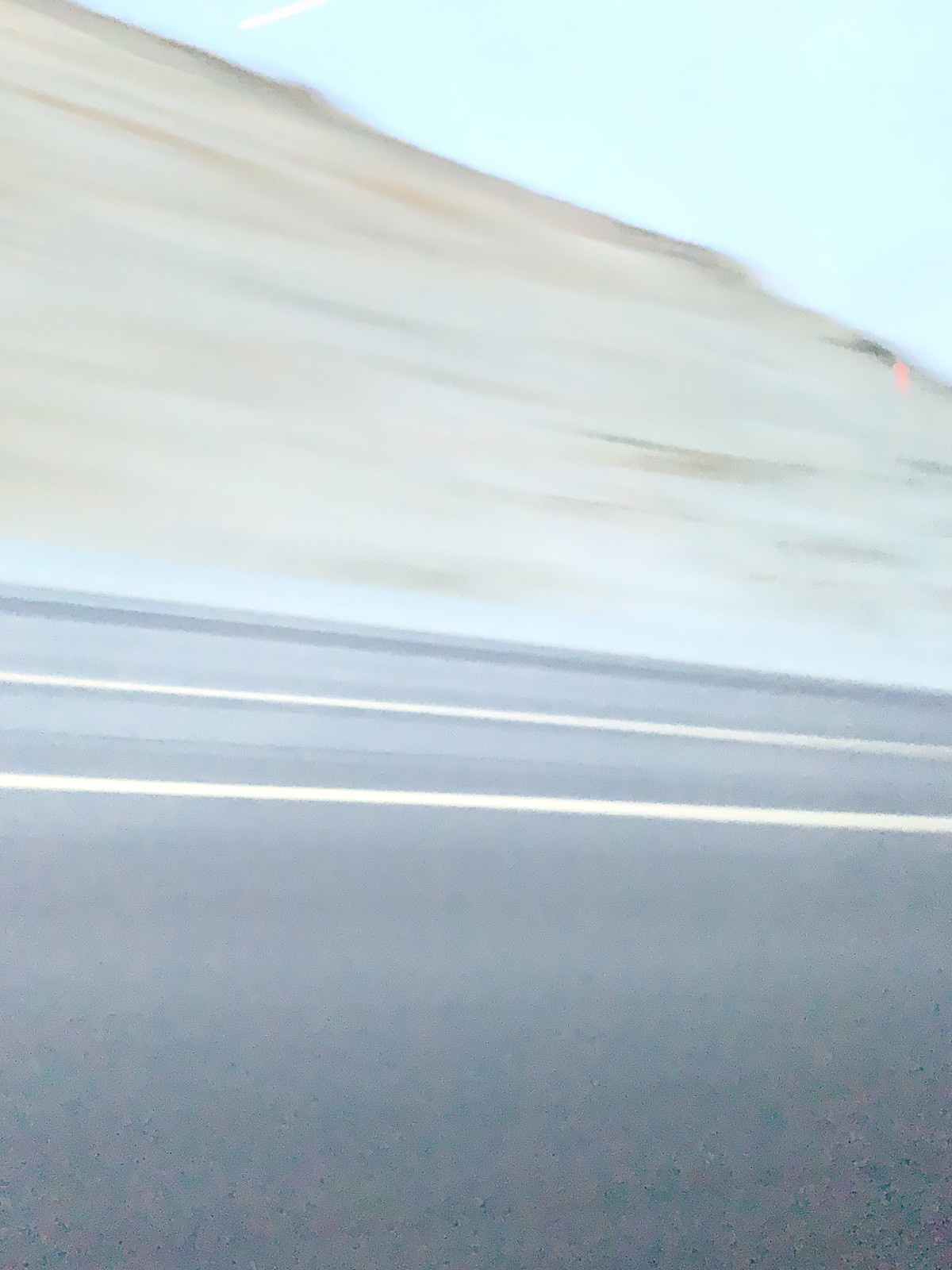A vertical artwork, potentially a painting, captures a serene landscape scene. The foreground prominently features a gray road with two white dividing lines, suggesting a freeway or major road. This road spans the middle to the bottom half of the image. Above the road, the landscape transitions to a tan-colored area with visible brush strokes, evoking the texture of a hillside. Crowning the horizon, a light blue sky completes the composition. The piece employs a muted, undersaturated palette of complementary colors, lending a tranquil and somewhat subdued atmosphere to the scene.